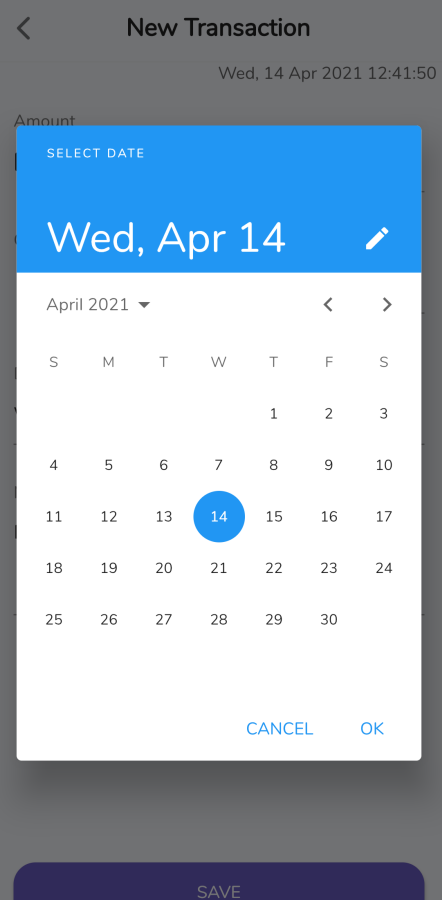The image depicts a mobile application's interface featuring a "New Transaction" screen. Most of the screen is currently obstructed by a pop-up calendar with today’s date highlighted as Wednesday, April 14, 2021. The calendar layout is standard, showing each week in rows starting from Sunday and ending on Saturday. 

In the background, slightly visible behind the pop-up, there is a prominent blue “Save” button, likely for confirming the transaction details once finalized. The main page itself remains hidden due to the pop-up, but it appears to be part of a process that involves scheduling a payment or transaction. There is a pen or pencil icon on the calendar, suggesting that users can add or edit events on specific dates. Both the main interface and the pop-up feature a clean, white background. Additionally, the interface shows the current time as 12:41:50.